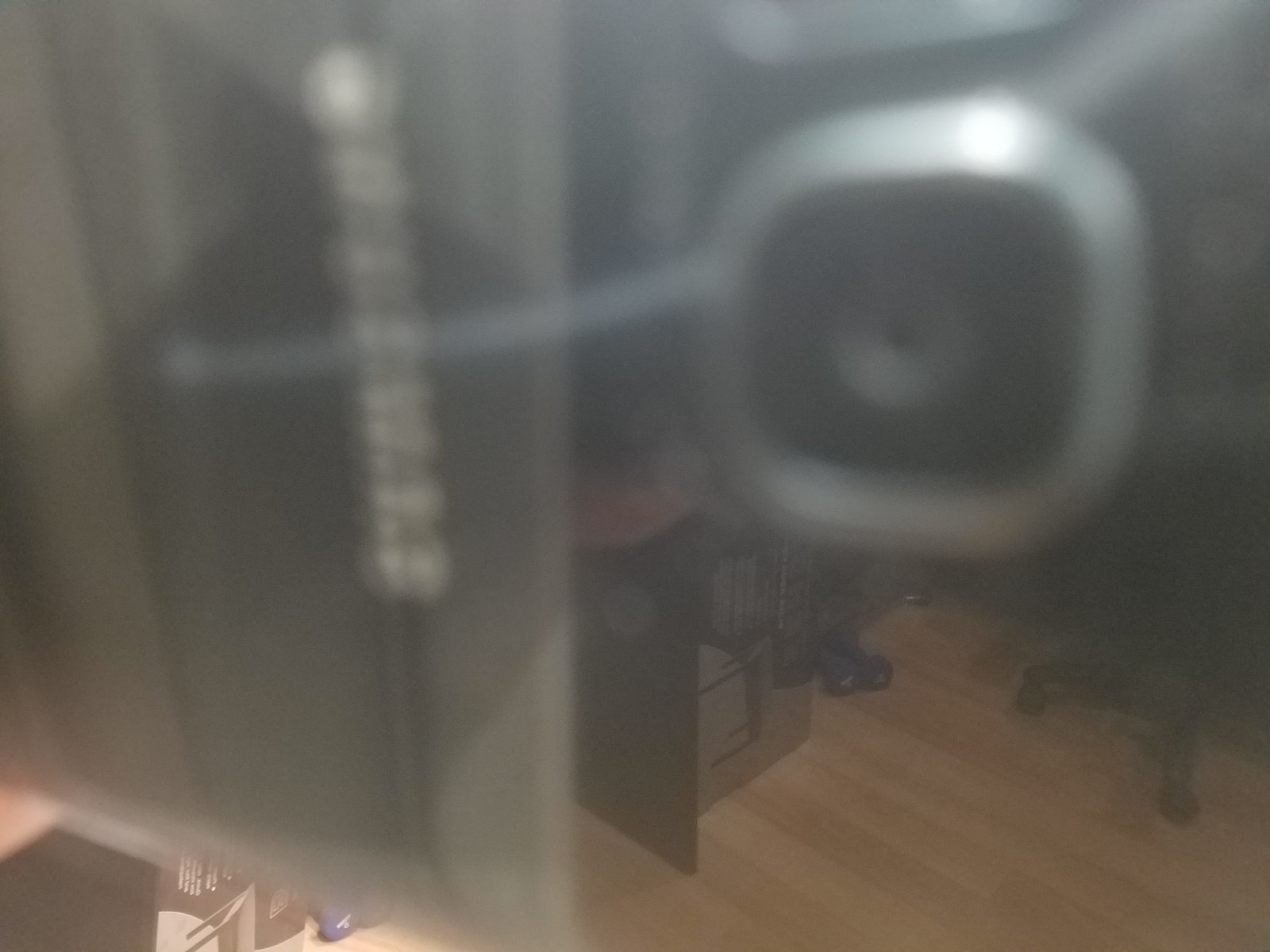A blurred photograph captures the interior of a house or apartment, seemingly taken from behind a TV or another piece of electronic equipment. In the upper right-hand corner, a black object with a front-facing square surrounded by silver chrome, possibly a speaker or remote sensor, catches the eye. To its left, another large, black rectangular object remains indistinguishable due to the obstruction. Despite these objects partially blocking the view, the light brown, wood-paneled floor beneath them is clearly visible. A pair of blue weights and the base of a silver chair can be seen in the background, adding a touch of domesticity to the scene.